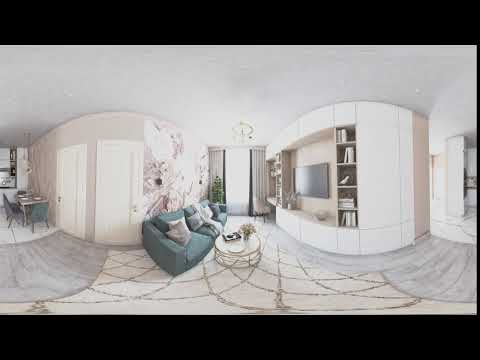In this image, taken during the daytime inside a home, we see a well-lit living room with a variety of elements meticulously arranged in a light, airy setting. The picture features a solid black border at the top and bottom, framing the scene. The floor consists of a light-colored wood with a white rug featuring a gray checkerboard pattern, centrally situated beneath a white and gold circular coffee table adorned with flowers and a book.

At the center of the composition is a dusty teal sofa, positioned against a white wall. The sofa is complemented by several light gray and white throw pillows. Facing the sofa, we see a wall-mounted TV flanked on the right side by narrow, inset shelves filled with white books and decorative items, and on the left side by two white doors. To the left of these doors stands a dinette table with chairs that match the color of the sofa, positioned near white curtained windows. The overall color scheme of the room includes shades of white, off-white, tan, green, and brown, creating a cohesive and inviting atmosphere. The slight curvature observed in the image hints at the use of a fisheye lens, adding a unique perspective to the room.